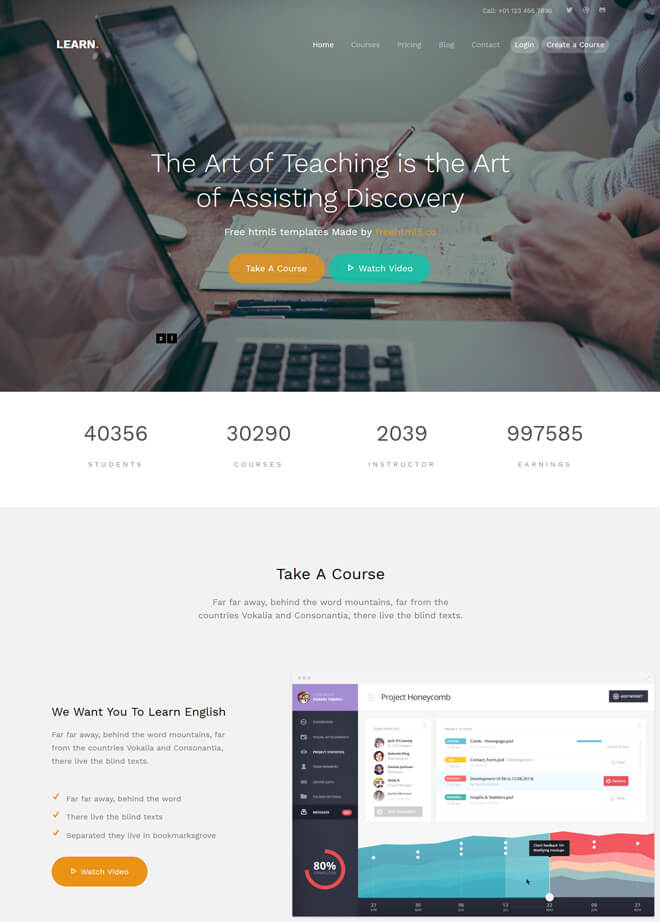The image displayed is a comprehensive view of a web page, divided into two sections, top and bottom. At the top, the word "Learn" is prominently featured in bold white text, set against a slightly faded background showcasing a collaborative setting. The background image captures a clear view of two laptops placed on a table, partially obscured by the two individuals present in the scene. Only the hands and forearms of these individuals are visible, indicating they are engaged in an activity, possibly drawing or taking notes with the pens they hold. Two additional pens rest on the table. One person wears a long-sleeved business shirt, suggesting a formal work environment.

Below this visual depiction, statistical data is presented in a structured format. It lists "40,356" under the label "students," "3,290" under "courses," and "2,039" under "instructors." This information denotes the scale and breadth of the platform’s user base and offerings.

In the lower section of the page, a call-to-action message reads "Take a Course," adjacent to a visual associated with "Project Honeycomb." On the left side, accompanying text urges readers to "We want you to learn English," followed by additional details and a button inviting viewers to watch a video for more information.